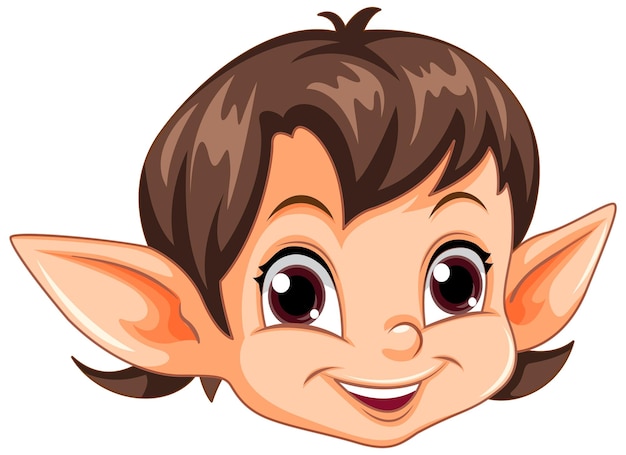This is a detailed, colorful, children's style drawing of an elf-like animated character's head and face. The elf has medium-length brown hair styled in a short pixie cut with two slightly spiky tufts protruding from the top. The hair also extends just below the large, pointed elf ears that jut out prominently from either side of the head. The elf has a happy, expressive face with thin, curved brown eyebrows that emphasize the joy in its eyes. Sparkling reflections highlight the large, brown eyes with black pupils, adding to the overall cheerful expression. The elf's face is a medium light tannish-peach color, and it features a small button nose. A big smile reveals white teeth, and the inside of the mouth is colored brownish-red. There is no background or visible body, focusing all attention on the endearing, up-close facial details.